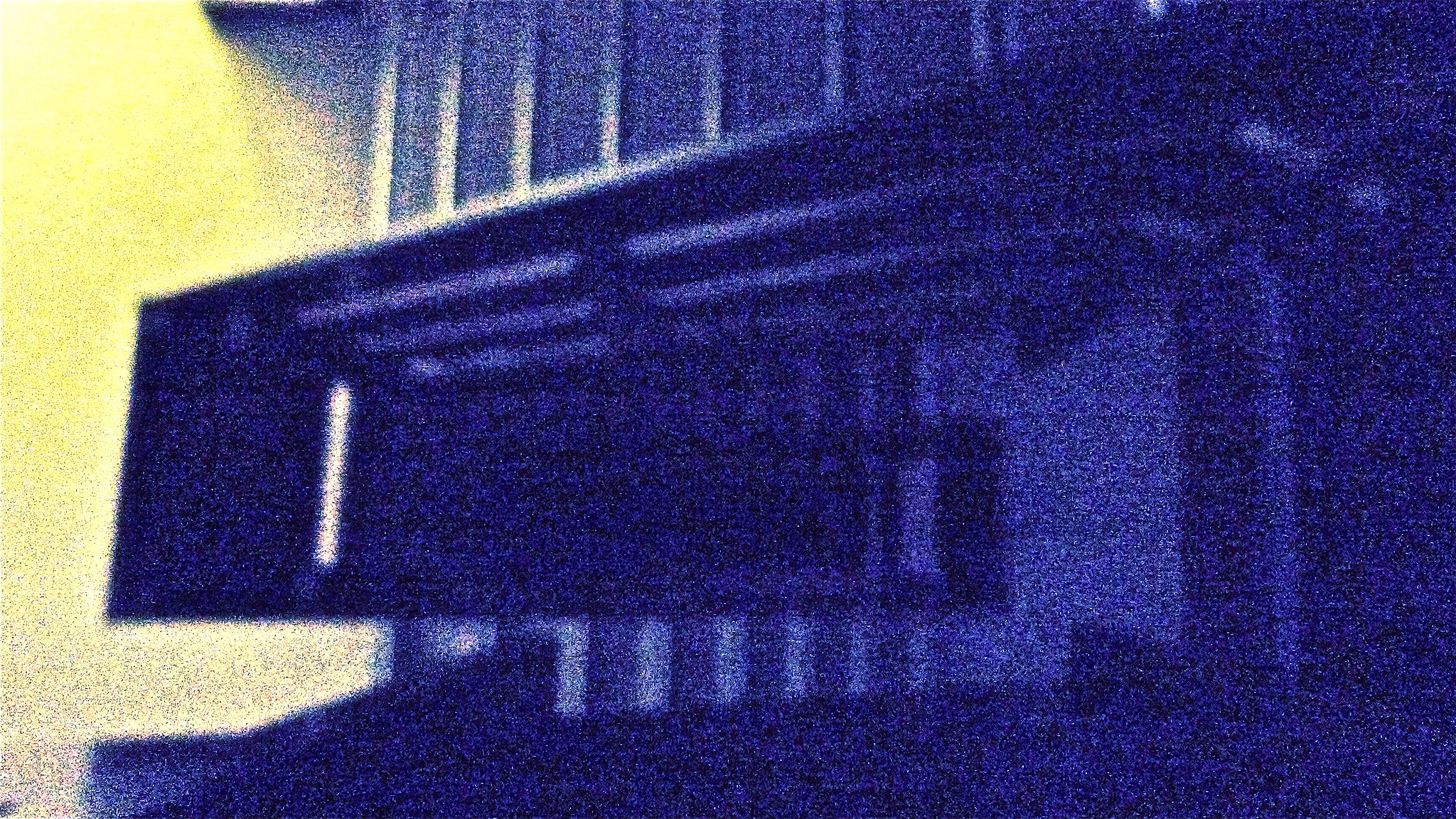The image depicts a dimly lit, grainy scene with noticeable white speckles, contributing to its grainy texture. Dominating the left-hand side is a large, distinctly yellow section, possibly indicating the side of a building. Extending from this structure is an awning, characterized by side panels that descend halfway down, each featuring small openings. The awning construction comprises roughly four boards, which seemingly draw closer to the camera. The overall composition suggests an obscured view of an architectural element, shadowed in darkness.